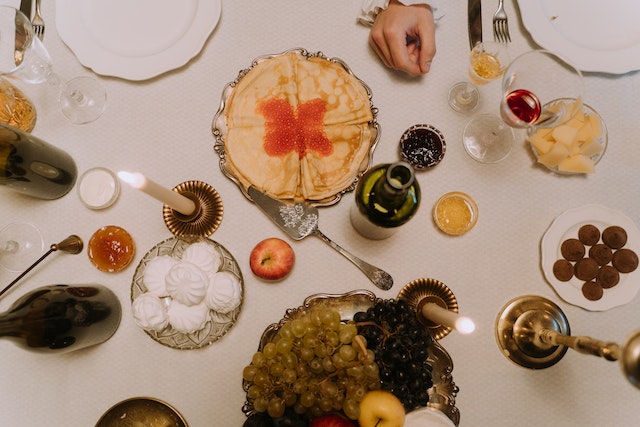In an overhead image taken from a landscape perspective, we see a beautifully set table adorned with an array of dishes and drinks placed on a white tablecloth, likely for a family gathering or a deck event. Dominating the center, there's a Caucasian hand with a white, ruffled sleeve, reaching into the scene. Surrounding this hand, to the right, are a fork and knife alongside a textured ceramic plate. There’s a striking arrangement of food and drink: a glass with a light yellow liquid, a goblet with red wine, and an adjacent plate topped with light yellow items. Directly below the hand, a glass filled with what appears to be black jam sits next to a plate featuring four slices of a pie adorned with orange dots, possibly caviar on bellinis. A silver pie cutter lies nearby. There’s also an array of fruit including a yellow apple and another plate filled with white balls that resemble macaroons or meringue cookies.

To the bottom right of this setup is a fruit bowl featuring grapes and another candle. Clear wine glasses, both empty and partially filled with light red wine, are scattered across the table. Adding to the festive spread, there are additional wine bottles, some smaller clear glasses with an orange liquid, and several plates with dark brown, small cookies. The scene includes white candles with brass bases, providing a warm, inviting ambiance. The overall presentation is elegant, hinting at a celebratory or special occasion.